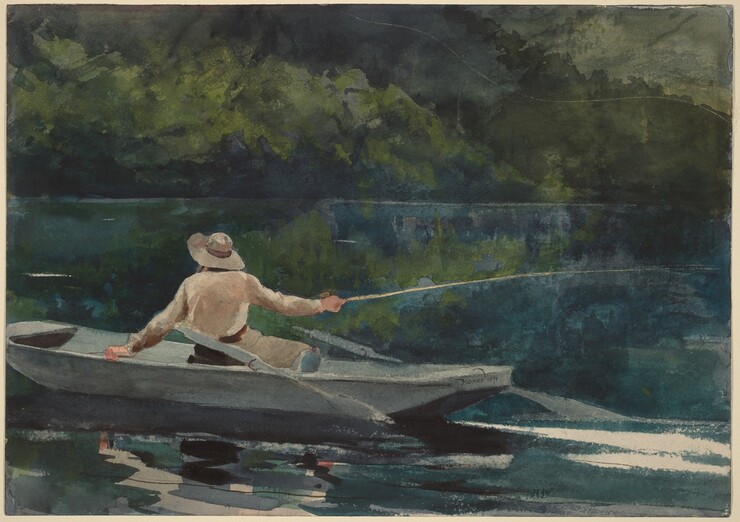In this serene, rectangular watercolor illustration, a solitary figure is depicted in the center of the composition, seated in a small, gray-hued rowboat amidst a tranquil lake. The water, showcasing clear blue tones, reflects the verdant foliage and wooded area that form the backdrop. The figure, whose back is turned towards us, is attired in a wide-brimmed fisherman's hat and a long-sleeved shirt paired with pants. This person is in the midst of fishing, holding a fishing rod extended outward, poised to cast. The calm, reflective surface of the lake transitions subtly to lighter, white hues near the boat, enhancing the overall softness and muted color palette of the scene. Delicate details like branches hanging over the water and the interplay of green and blue hues contribute to the painting’s peaceful and immersive atmosphere.